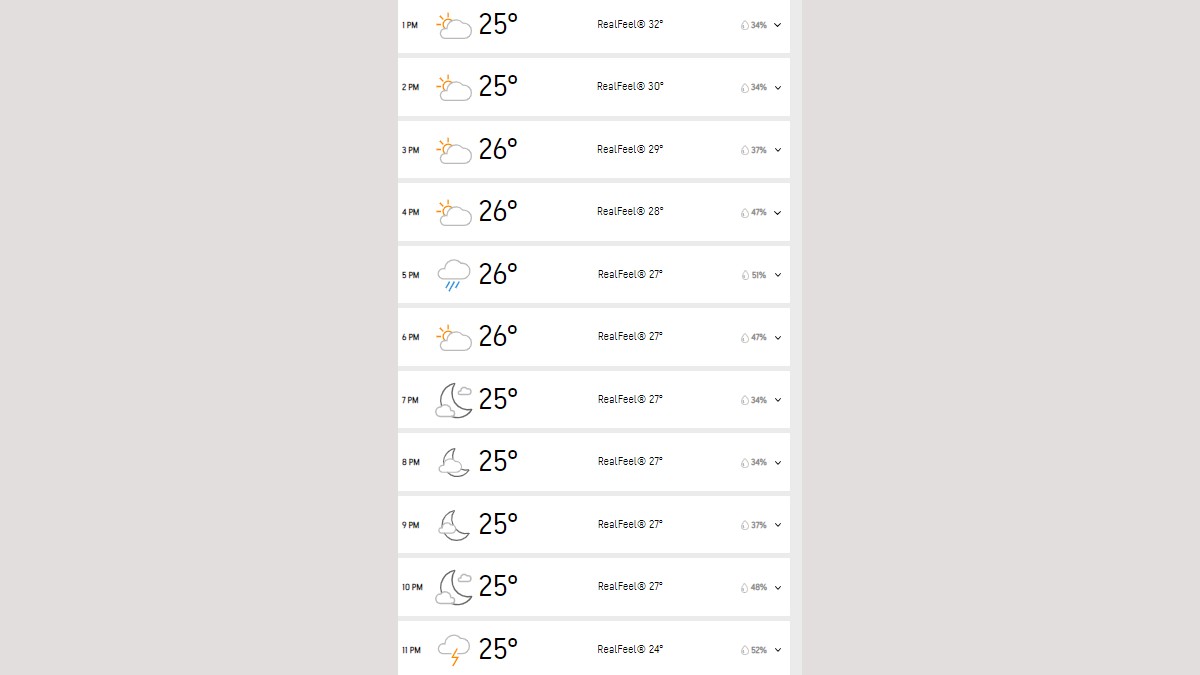This is a cropped and edited screenshot of a mobile weather app displaying hourly forecasts arranged vertically. At the top, the entry for 1 PM is shown, featuring a weather icon with a cloud and sunray, indicating partly cloudy skies. The temperature is indicated as 32°F with a real-feel temperature nearby, and a humidity level listed as 34%. 

The next entry for 2 PM shows a similar format with a temperature of 25°F. Each subsequent hour—3 PM, 4 PM, 5 PM, 6 PM, 7 PM, 8 PM, 9 PM, 10 PM, and finally, 11 PM—follows the same structure: the time appears on the left, the weather condition icon in the middle, showing varying degrees of cloudiness and sun, and a dropdown box on the far right displaying the probability of rain with a percentage.

The detailed design of the app provides a clear, hour-by-hour outlook, making it easy to see how the weather changes over the course of the day, with 11 PM being the final forecast entry at the bottom of the screen.